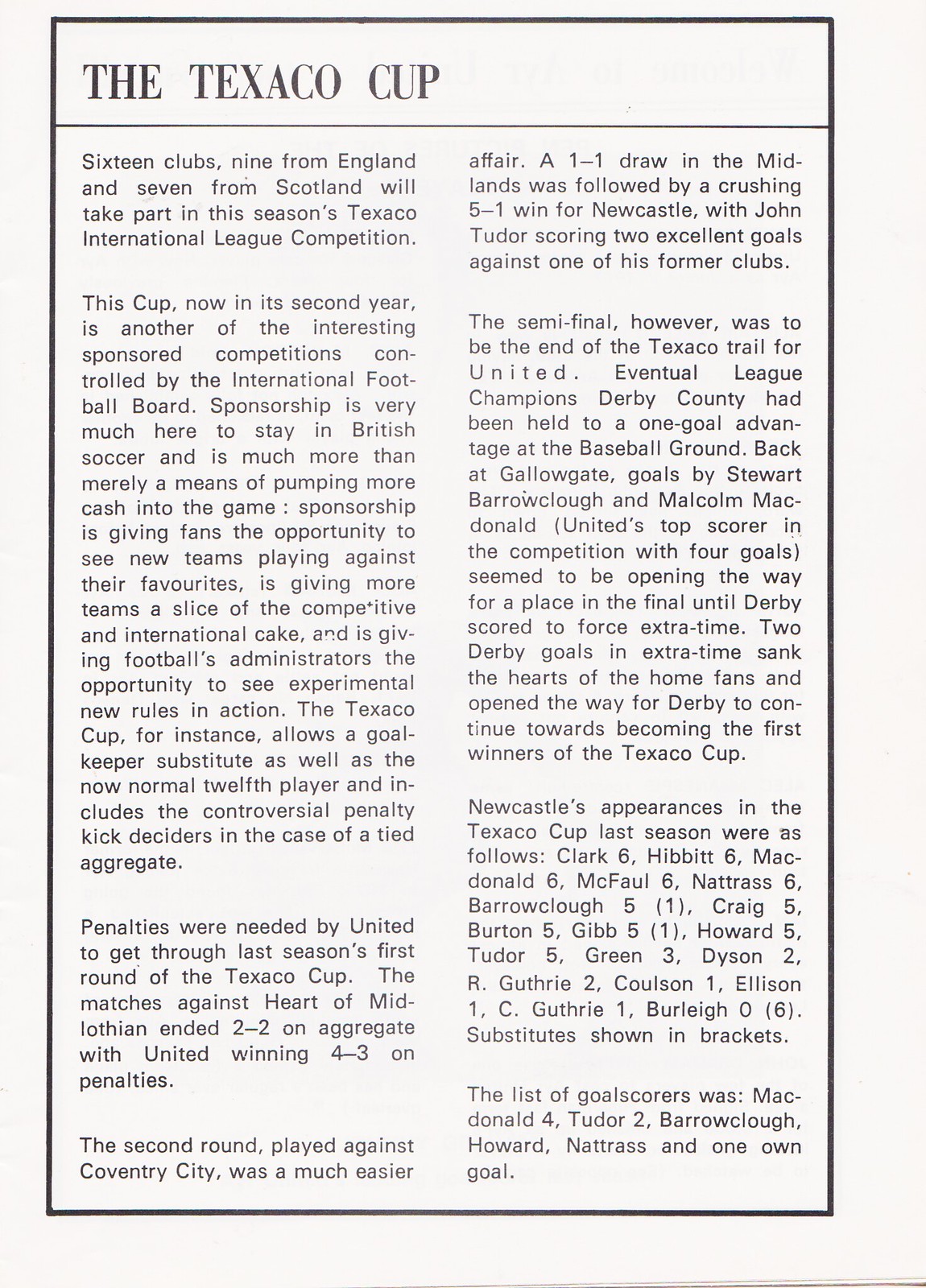A black and white newspaper clipping titled "The Texaco Cup" announces that 16 clubs, comprising 9 from England and 7 from Scotland, will compete in this season's Texaco International League competition. This cup, now in its second year, is sponsored by the International Football Board, highlighting the growing significance of sponsorship in British soccer. Sponsorship is not just about injecting more funds into the game but also about providing fans the chance to see new teams play against their favorites, giving more teams competitive exposure, and allowing football administrators to test new experimental rules. The Texaco Cup includes special provisions, such as allowing a goalkeeper substitution and the use of penalty kick deciders in case of a tied aggregate. 

Last season, penalties were required for United to advance past the first round against Heart of Midlothian, with the aggregate score tied at 2-2 before United edged through with a 4-3 penalty shootout victory. The second round saw United ease past Coventry City with a 1-1 away draw followed by a dominant 5-1 home win, featuring two goals by John Tudor against his former club. Despite this success, United's journey ended in the semi-final against Derby County. After a narrow one-goal deficit from the first leg, hopes soared as Stuart Barrowclaw and Malcolm McDonald scored at Gallowgate. However, Derby equalized to force extra time and then sealed their victory with two additional goals, eventually becoming the cup’s first winners.

Newcastle’s player appearances in the Texaco Cup were listed as follows: Clark 6, Hibbett 6, McDonald 6, McFall 6, Natris 6, Barrowclaw 5, Craig 5, Burton 5, Gibb 5, Howard 5, Tudor 5, Green 3, Dyson 2, R. Guthrie 2, Colson 1, Ellison 1, C. Guthrie 1, Burleigh 0 (substitutes in brackets). The goal scorers included McDonald with 4 goals, Tudor with 2, followed by Barrowclaw, Howard, Natris, and one own goal. This page, seemingly clipped from the left half of a magazine, provides a detailed account of the Texaco Cup's competition and significance.